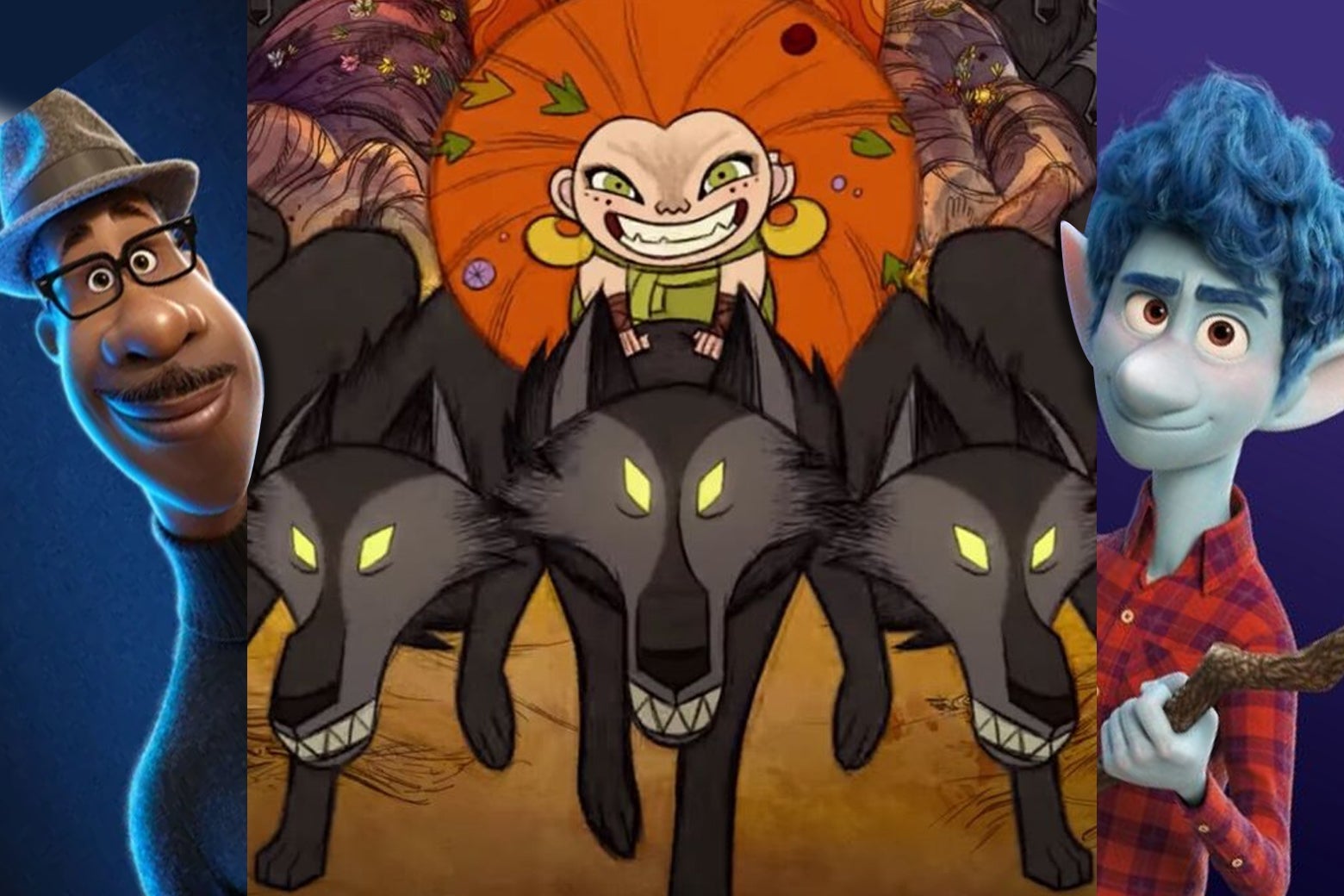This image, possibly a still from an animated movie or perhaps used as a thumbnail for a YouTube video, features a vibrant and dynamic 2D illustration in its center. Dominating the scene are three black and gray wolves with piercing yellow eyes and bared menacing teeth, arranged with one in the middle and two flanking it. Riding atop the central wolf is a lively girl with a massive, circular, bushy orange-red hair that spreads out behind her almost like a saucer. She sports a green tunic, sparkling green eyes, yellow earrings, and a wide, somewhat mischievous grin. 

Flanking the central image on either side are more realistically rendered characters: on the left, there's a man with glasses, a mustache, a detective-style hat, and a cautious demeanor as he peeks into the frame. On the right is a blue-skinned, blue-haired man, dressed in a red flannel shirt, holding a stick, resembling an elf-like character. This juxtaposition of artistic styles hints at a playful, adventurous theme typical of Disney-like animated movies.